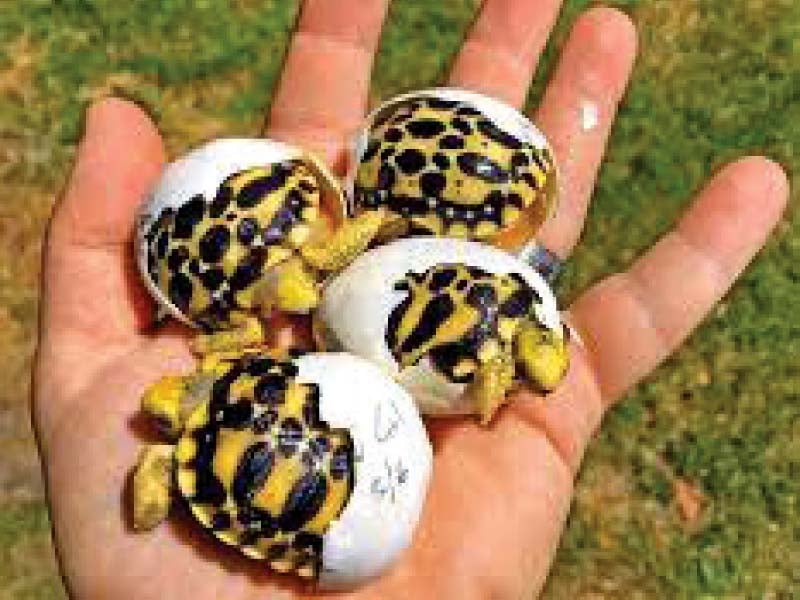In this somewhat blurred and pixelated image, a close-up view of a light-colored left hand, palm side up with fingers splayed, dominates the frame. A silver ring is visible on the ring finger of the hand. Nestled in the palm are four yellowish green baby turtles, each with distinctive black markings and partially encased in their white eggshells. Behind the hand, a grassy background can be seen. The turtles, facing in various directions, display their tiny heads and limbs as they emerge from their shells.